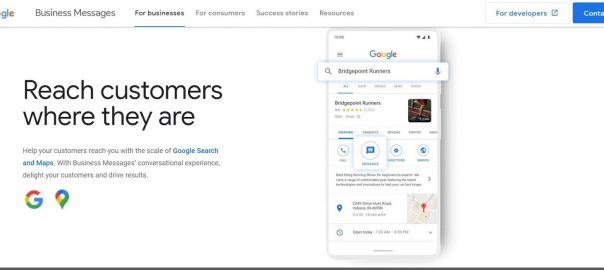The image showcases a webpage with a navigation bar at the top featuring five categories: "Business Messages," "For Businesses," "For Customers," "Success Stories," and "Resources." The "For Businesses" category is highlighted in a bold font with a blue underline, indicating it is the currently selected section. Below the navigation bar, a prominent heading reads, "Reach customers where they are. Help your customers reach you with the scale of Google Search and Maps," with "Google Search and Maps" emphasized in blue while the rest of the text is in gray. Further down, there are bullet points listing "Business messages," "Conversational experience," "Delight your customers," and "Drive results."

On the left side, recognizable icons of Google's services are displayed: the "G" logo for Google and the pinpoint icon for Google Maps. To the right, there is a screenshot of a Google Search result for a place named 'Bridge Points.' Although the text is blurry, the search result clearly shows typical Google elements such as star ratings and a map location.